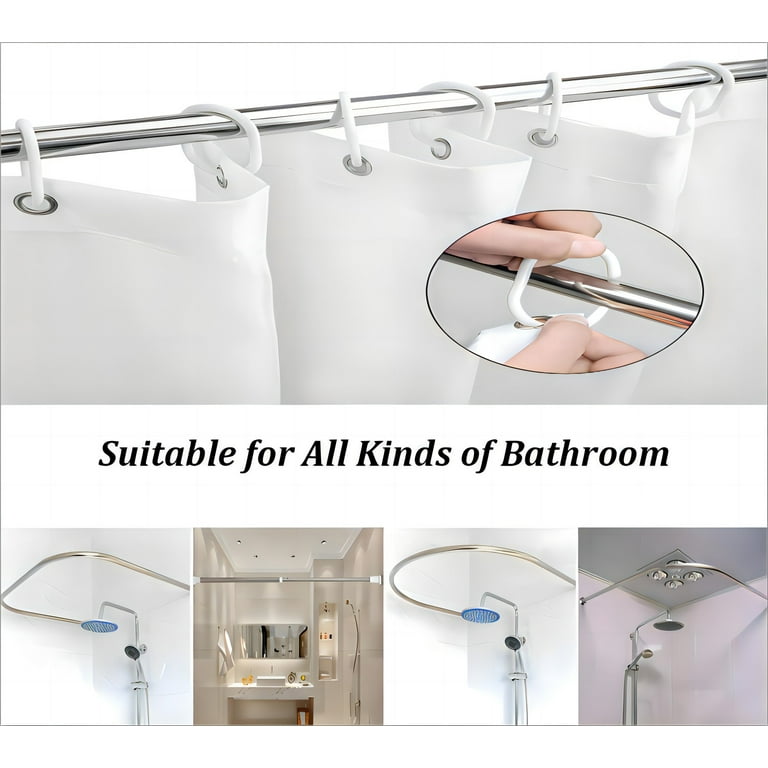The image features the upper part of a bathroom shower curtain setup. At the top, a shiny silver stainless steel rod runs horizontally. A white shower curtain is hung on this rod, adorned with multiple white rings. On the bottom right, there's an inset oval showing two human hands affixing the white rings onto the rod. The image also includes a black italic title that reads, "Suitable for all kinds of bathrooms." Beneath this are four smaller images displaying diverse configurations of stainless steel rods: rectangular, strictly horizontal, curved, and triangular shapes, each placed in different bathroom settings.